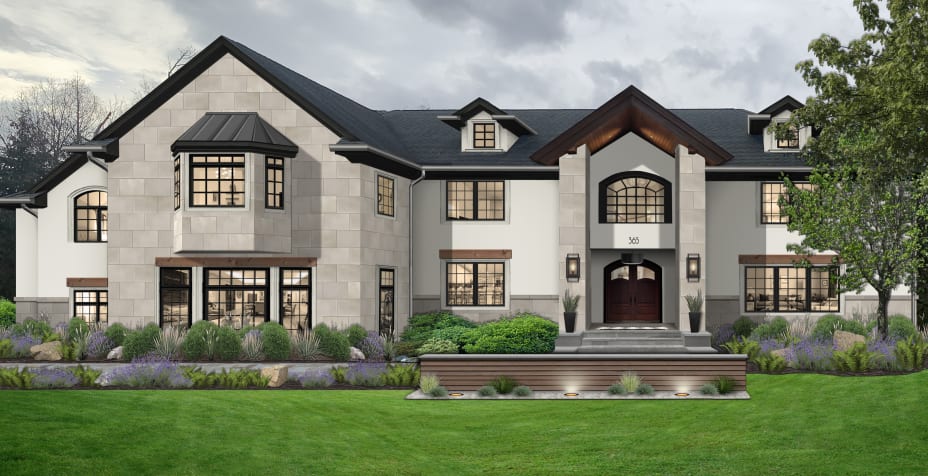The image depicts a large, gray-stone mansion, possibly created through computer design, blending a realistic and slightly artistic appeal. The mansion stands tall with at least two, possibly three floors, including an attic-like third floor with windows jutting out from the dark gray, charcoal-colored roof. The exterior of the house features a combination of gray stone blocks and white accents, creating a distinguished look. The roof is dark gray, almost black, with additional small, roofed sections over some windows.

At the forefront, there are two substantial brown, partially see-through entry doors beneath a prominent portico supported by stone columns. The overall design gives the appearance of a grand, expansive residence with multiple sections, including a square, angular front part that projects outward on the left side and another even section further back.

The meticulously maintained green lawn is accentuated with shrubs and small trees, particularly on the right side, some of which still have their leaves, suggesting a season transition. A set of stairs and a small brick wall lead up to the entrance, while a driveway extends on the left. The presence of outdoor lights around the grassy area and entrance hints at the onset of evening amidst an overcast gray sky, adding to the serene and somewhat dramatic atmosphere of the scene.